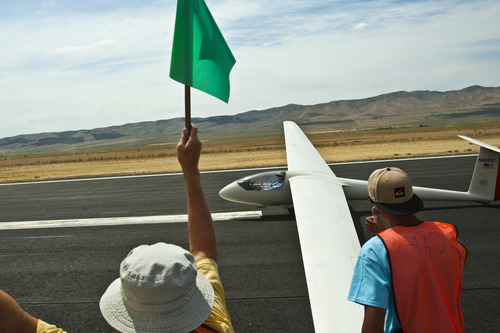This photograph captures a sunny, outdoor scene at an airport runway situated in a desert landscape. In the foreground, two individuals are seen from the back. The person on the left is wearing a white bucket hat and has their arm raised, holding a green flag, as if signaling for an event to start. Their other arm hangs at their side. To the right stands another person dressed in a turquoise blue shirt, an orange safety vest marked with "CAF," and a tan baseball cap worn backwards. This individual appears to be giving a thumbs-up gesture towards the pilot in the nearby small white glider, which is positioned on the runway's center line and readying for takeoff. The runway itself is asphalt with a white stripe indicating the center line. In the background stretches a vast, sandy terrain leading up to a distant tan-brown mountain range under a partly cloudy blue sky. The predominant colors are black, white, orange, blue, green, and various sandy hues, contributing to a vivid and dynamic atmosphere.